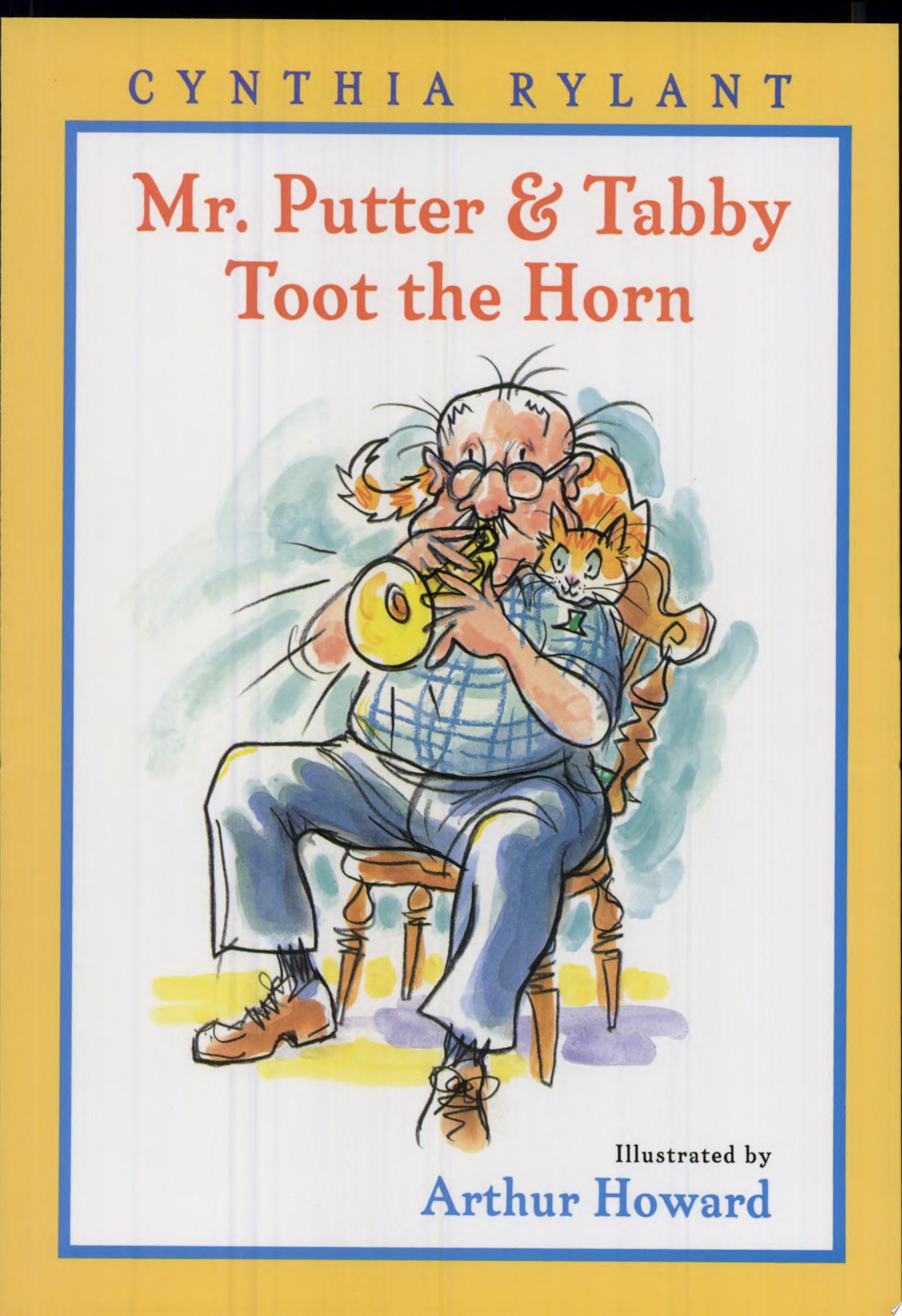This is an illustration from a children's book cover titled "Mr. Putter and Tabby Toot the Horn" by Cynthia Rylant, with illustrations by Arthur Howard. The image features an elderly, bald man with squiggly eyebrows and glasses sitting on a brown wooden chair. He is wearing a white and blue plaid shirt, blue pants, and brown shoes, while blowing a shiny yellow trumpet. An orange and white striped cat, Tabby, sits calmly on his shoulders. The background of the illustration is white, surrounded by a blue border, which is further enclosed by a yellow border. Within the yellow border, at the top center, is Cynthia Rylant's name in uppercase blue letters. The title of the book appears in red text above the man, and the illustrator's name, Arthur Howard, is written in black and blue text in the lower right-hand corner. The overall design evokes a whimsical, cartoony feel reminiscent of coloring or comic pages in a newspaper.